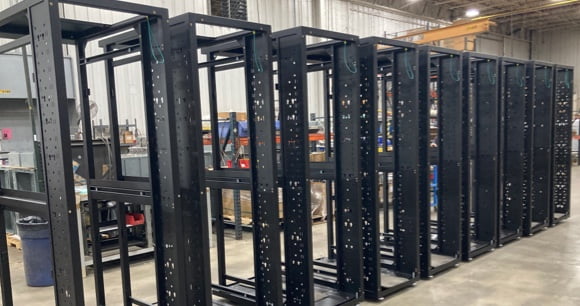The image appears to be inside a large, well-lit factory or industrial workshop with gray concrete floors and high ceilings. It shows a row of approximately nine or ten tall metal frames, resembling old-fashioned payphone booths or metal detectors, though they lack glass and are more sturdy and rectangular. These frames are deep black or dark metal, with holes possibly for ventilation or visibility, and they seem to have casters on the bottom for mobility. The frames are arranged in a neat line, slightly angled, and you can see a blue garbage can positioned on the left side of the image. The background features a workshop setting, with metal walls and a window. The various colors present include black from the frames, and shades of white, orange, red, yellow, and blue from different equipment and objects scattered around. There is no visible text or any people or animals in the scene. The overall look gives an impression of an organized yet busy industrial workspace with vintage elements.